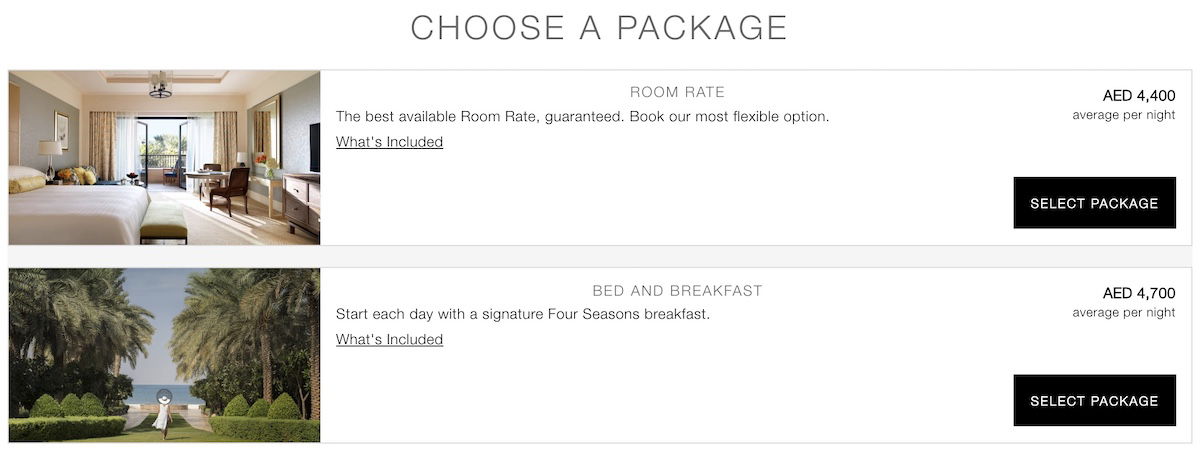Screenshot Caption:

The screenshot showcases a webpage offering two luxurious accommodation packages at a beautiful hotel. The first option, featured prominently, is a spacious and elegantly designed hotel room. The room boasts French doors that open to a balcony area, revealing a picturesque seating area. Inside, the room is furnished with a large, plush bed accompanied by a seating bench at its foot, a dresser topped with a TV, and a mirror on the wall. The room rate is described as the best available rate, accompanied by a clickable link for more details on what's included, and it is priced at AED 4,400 per night. A black button labeled "Select Package" allows guests to proceed with booking.

The second option available is a bed-and-breakfast package. The accompanying image depicts a serene scene of a woman walking towards a beach, flanked by beautiful palm trees and decorative bushes, creating a natural gateway to the sandy shores and open sea. This package promises to start each day with a signature Four Seasons breakfast and is listed at an average of AED 4,700 per night. Like the hotel room option, it has a black "Select Package" button for easy booking.